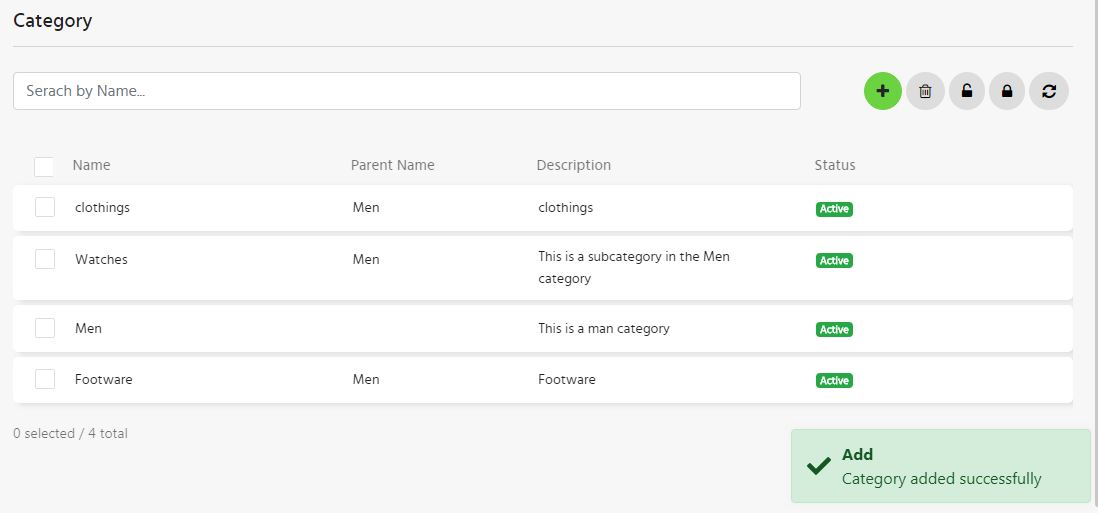The image displays a horizontal rectangular interface with a light gray-blue background. At the top left corner, the word "Category" is written in black text. Below this, a pale gray line runs horizontally across the screen. Beneath the line is a long white search bar, which contains the misspelled placeholder text "serach by name." To the right of the search bar, there is a black plus sign inside a green circle, a trash can icon for deletion, and two padlock icons—one unlocked and one locked. There is also a refresh symbol.

Below this toolbar, the left side of the screen features the word "Name" in light gray text with a checkbox next to it, followed by columns labeled "Parent Name," "Description," and "Status."

The first entry, displayed on a white banner, includes the word "Clothings" in gray text with a checkbox next to it. To the right, it lists "Men" under Parent Name, "Clothings" under Description, and a green box labeled "Active" under Status. 

The next entry also appears on a white banner and lists "Watches" with a checkbox next to it. Under Parent Name, it says "Men," and the Description reads "This is a subcategory in the men category." The Status column has another green box labeled "Active."

Following this is the entry for "Men," with no checkbox. The Description reads "This is a men category," and the Status column once again shows a green box labeled "Active."